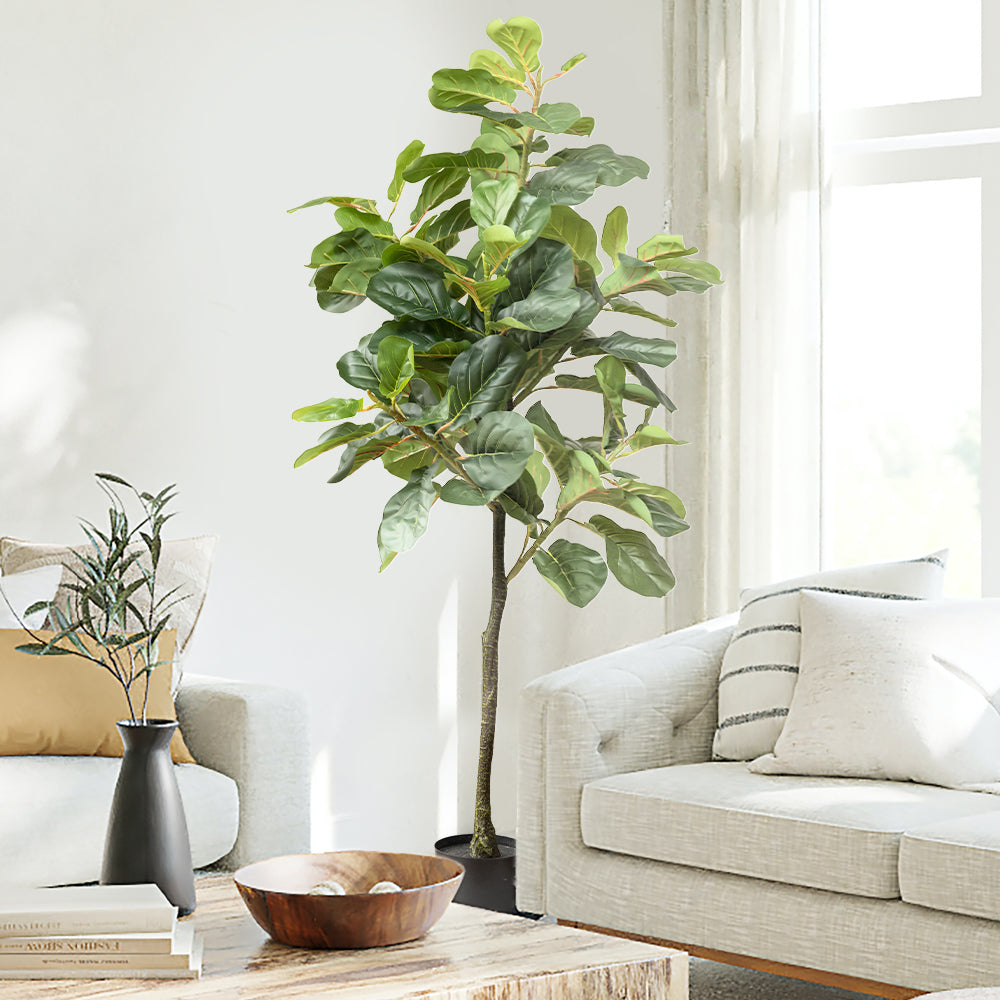The image captures a bright and clear living room corner, showcasing a well-lit, cozy space with white walls. On the right side, a light gray couch with a wooden brown base sits against a large window adorned with white curtains. The couch is neatly decorated with a black and white striped pillow, and a plain white pillow. Sunlight filters in through the window, adding a natural glow to the scene. At the center of the image stands a tall, potted plant with large green leaves, adding a touch of greenery to the room. Below, a wooden table occupies the lower left corner, featuring a wooden bowl, a black vase with more green foliage, and a stack of thin paperback books. Positioned toward the left side, a light gray chair or love seat with a yellow pillow and a gray pillow complements the overall aesthetic. The space is unified by a gray carpet visible beneath the couch, enhancing the warm and inviting atmosphere.